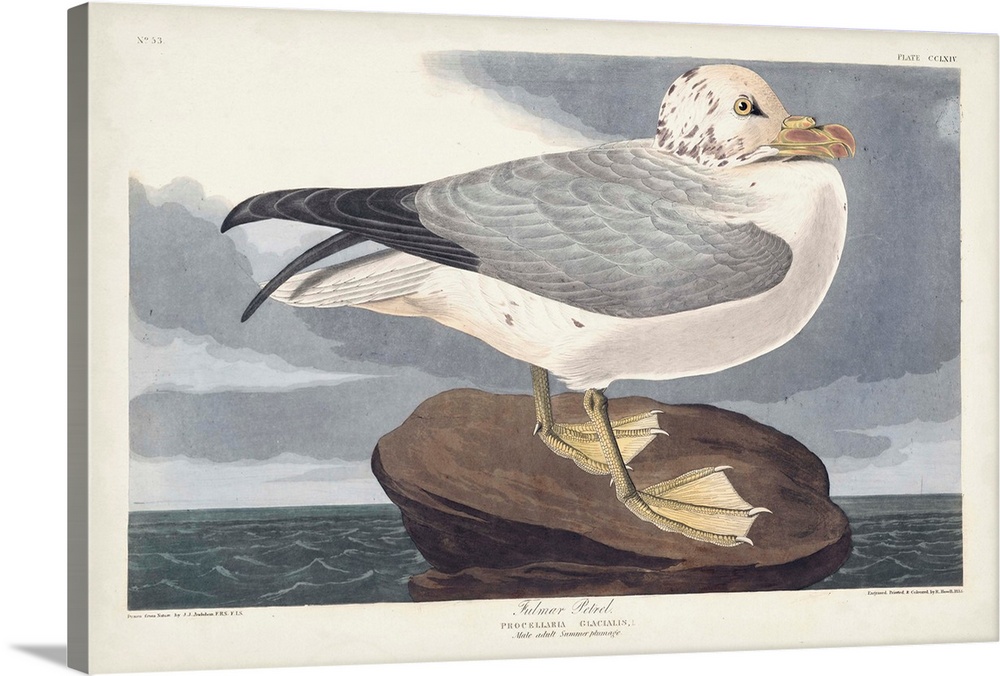The image depicts a painting or drawing of a large seagull-like bird, specifically a Fomar petrel, perched on a brown rock surrounded by a body of water. The bird has a white head and belly, a grey back, and darker tail feathers. Its beak shows distinctive yellow and reddish-pink coloration, and it has yellow, webbed feet that appear slightly scaly. The bird’s eye is yellow, framed by fine grey markings on the back of its neck.

In the background, there is a grey and white cloudy sky, with a dark sea beneath it. The painting is bordered by a cream-colored frame. The upper left corner of the frame is marked with the number 53, while the upper right corner says "plate CCXIV". Text along the bottom edge of the painting includes the bird's scientific name, "Priscilla Eris, Glacialis," and "Fomar petrel," though some of the text is difficult to read due to its small size. The painting, which may be a stock image or part of a collection, is presented in a way that suggests a 3D frame, offering a realistic perspective of how it might look if displayed.